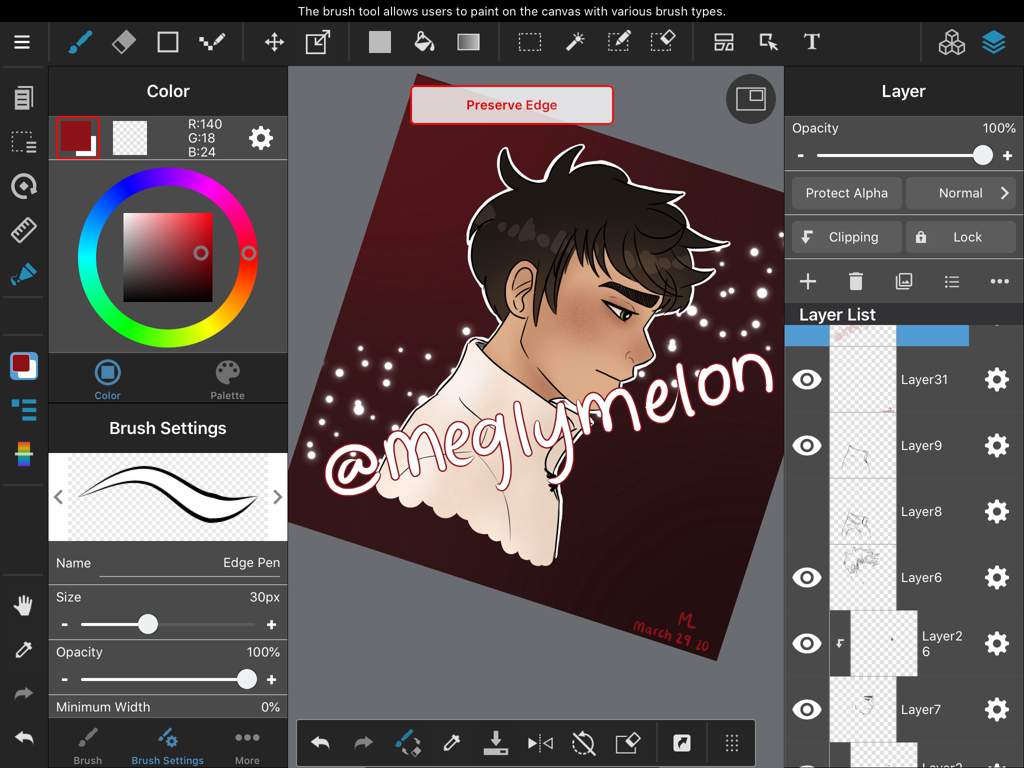This image is a detailed screenshot of a painting application displayed on a computer screen. At the very top, there is a notification that reads: "This brush tool allows users to paint on the canvas with various brush types." The top menu includes multiple options, and there are additional tools on either side of the interface.

In the center of the canvas is a square area colored in burgundy, showcasing a cartoon illustration of a man. The man is depicted looking to the right, with brown hair and thick brown eyebrows. He is wearing a white shirt, and a pattern of white dots surrounds him. Overlaying the illustration are the words "at Magli Mellon" and at the bottom in red text, it reads "ML March 29th 20."

To the left of the central image, there is a color wheel for selecting hues, alongside brush settings and size adjustment options. On the right side are various layer management tools labeled as follows: "Layer," "Protect Alpha," "Normal," "Clipping," and "Lock." There is also a plus sign icon for adding layers, a trash can icon for deleting layers or items, and a picture icon. Below these icons is a list indicating the current layers being worked on.